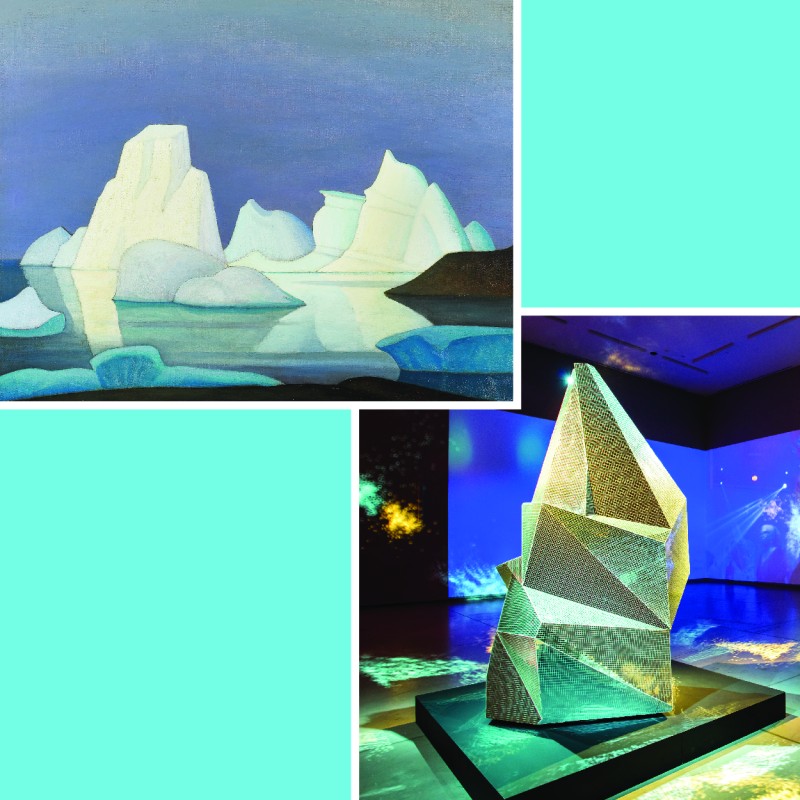The image is composed of four sections arranged in a square layout on a teal background. The top left section features a painting of icebergs floating on water, with hues of blue, green, and white under a hazy blue sky. Shadows accentuate the white and blue icebergs, which have greenish tints. The bottom left and top right sections are plain turquoise squares with no additional details. The bottom right section shows a sculpture displayed in a museum, placed in front of a dark blue screen. The sculpture, which suggests the form of an iceberg, is illuminated with turquoise and hints of yellow-gold lighting.